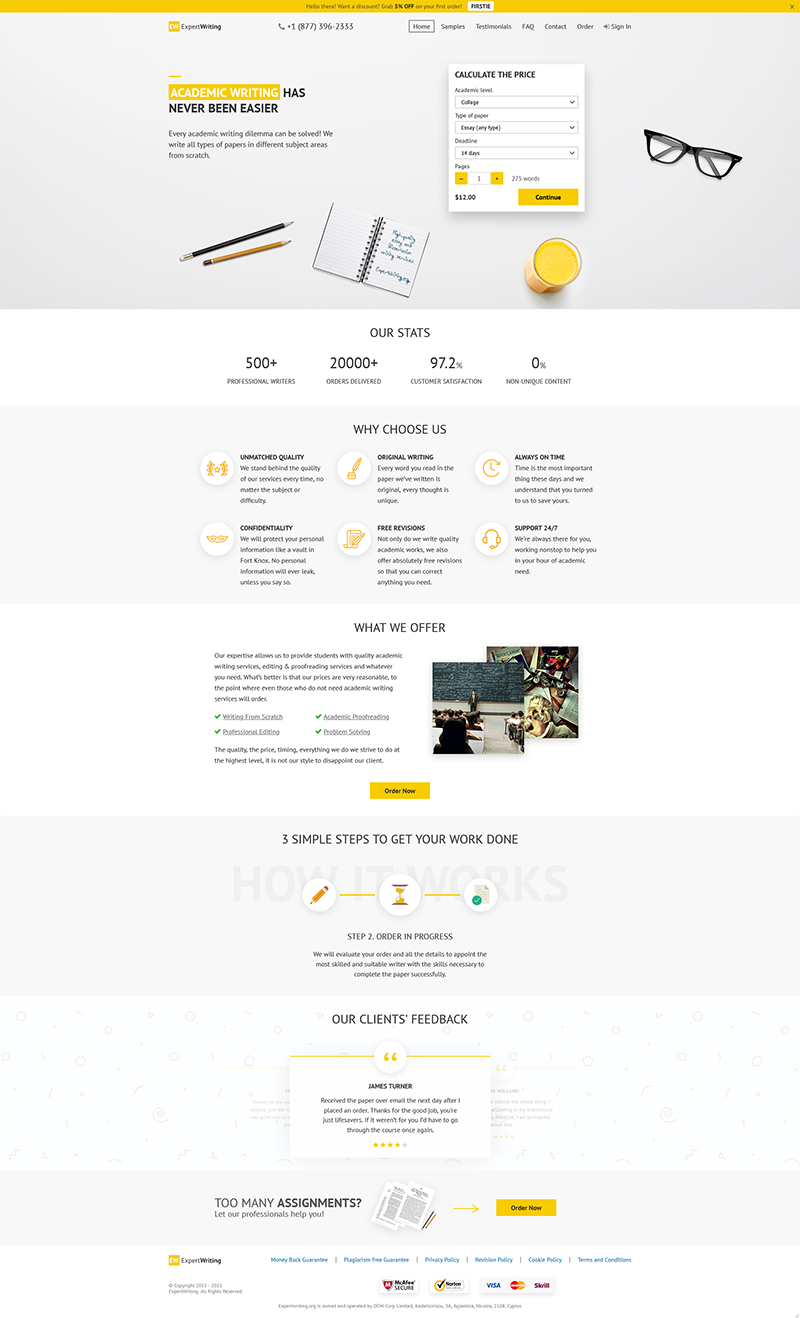The image depicts a compacted, busy webpage designed for a service specializing in professional and academic writing. The page is densely filled with text and graphics that are difficult to read due to their small size. The website features a clean layout with alternating light gray and white sections, each containing different types of content. 

At the top, there are clear navigation tabs labeled "Home," "Samples," "Testimonials," "FAQ," "Contact," "Sign In," and "Order." Below these tabs, various banners and text blocks populate the screen, including a section promoting "Academic Writing made Easy" and a small interactive calculator for users to estimate the price based on the number of days they need for completion.

The imagery includes visuals of common writing tools such as glasses, pens, pencils, and notepads, evoking an academic and professional atmosphere. A notable statistic highlights "500+ professional writers," indicating that the service employs human writers to complete assignments.

Further down, the webpage outlines a simple three-step process to get work done, paired with sections like "Our Client's Feedback" and prompts addressing issues like "Too many assignments?" suggesting the service caters primarily to students and business professionals seeking writing assistance without the hassle of a complicated process.

Overall, this detailed webpage offers a streamlined writing service aimed at easing the workload of its users with accessible features and professional support.